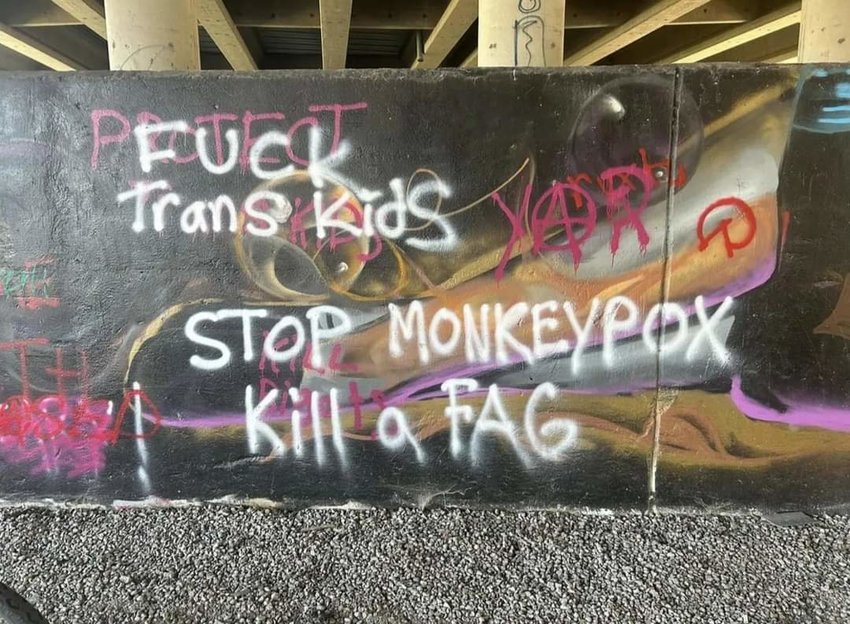The image is a detailed photograph taken during the daytime, showcasing a scene underneath a pier. It features three wide vertical columns that support the wooden planks forming the pier above. The ground is covered with gray gravel. Prominently displayed in the foreground is a black-painted wall defaced with graffiti in various colors, including white, pink, and red spray paint. 

The graffiti includes highly offensive and profane messages. In the upper left-hand corner, pink spray paint spells out “Protect kids,” which is overlaid by white spray paint reading, “Fuck trans kids.” Below this, further white spray paint messages include, “Stop monkey pox, kill a fag,” with additional pink spray paint seemingly stating, “Kill rights.” In the upper right-hand corner, someone wrote “Yar,” where the 'a' appears as an anarchy symbol.

Overall, the image paints a disturbing scene of vandalism and hate speech on a structure commonly found at a construction site or underneath a pier.